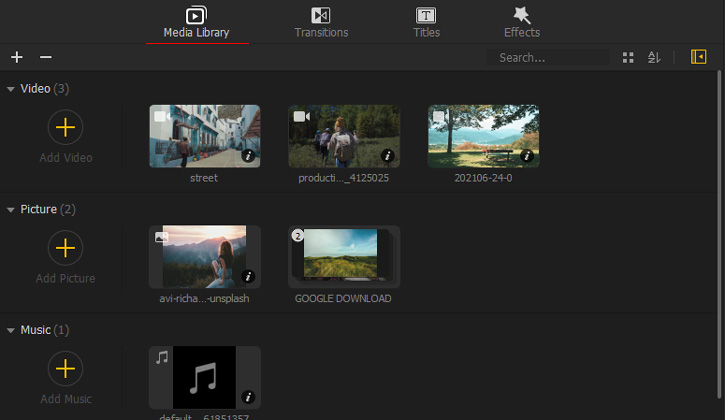A screenshot captures an intricate video editing software interface layout. At the top of the interface, there is a header featuring four menu options, each represented by unique icons: a play button for the Media Library, two touching triangles for Transitions, a capital 'T' for Titles, and a star with a wand for Effects. Directly beneath these menu options are plus and minus buttons situated on the left, and a search field on the right.

The interface showcases three distinct sections: Videos, Pictures, and Music. The Videos section includes a gray circle with a yellow plus sign labeled "Add Video," followed by thumbnails of three video clips on the right. Each thumbnail displays a video icon in the top-left corner. The video thumbnails are labeled "Street," "Production," and the third with just a date. The "Street" video depicts someone walking down a street bordered by blue buildings. The "Production" video shows people walking in a wilderness setting, and the date-labeled video features a park bench amidst a lush park.

In the Pictures section, there is also a gray circle with a yellow plus sign labeled "Add Picture," followed by two image thumbnails to the right. One thumbnail shows a woman gazing towards distant mountains, while the other appears to be an aerial shot of a landscape.

The Music section has a similar gray circle with a yellow plus sign, labeled "Add Music," and a field next to it displaying the word "default" with a light gray musical note icon overlaying a black square.

Overall, the screenshot provides a detailed look at the organized and feature-rich environment of the video editing software.